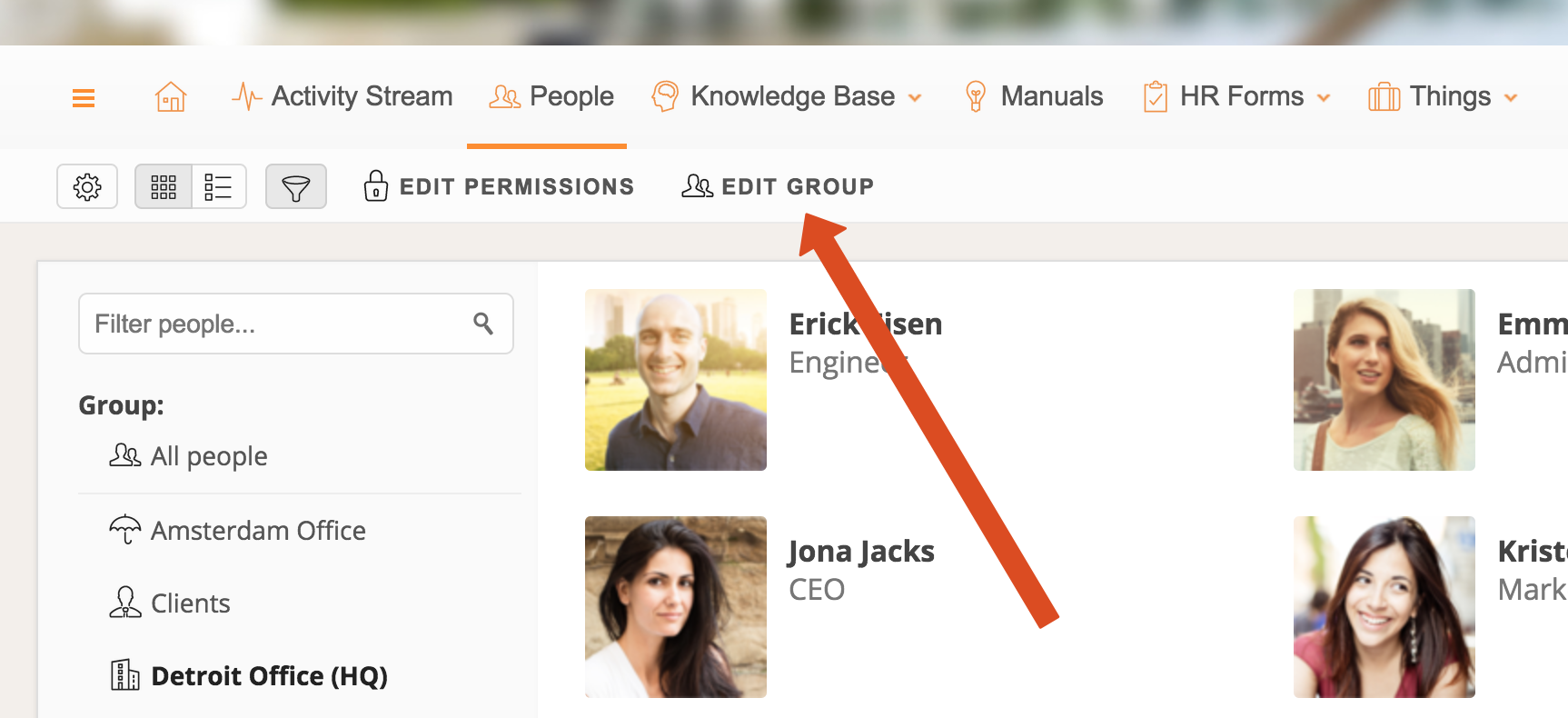In this image, we observe a professional interface with four profile pictures located at the bottom right. The central profile belongs to 'Eric,' who is identified as an Engineer. Eric appears to be a bald, white male wearing a blue shirt, depicted in a square-shaped photo. Below Eric’s picture is 'Jonah Jacks,' whose title is CEO. Jonah is a white individual with long black hair and is seen wearing a white shirt.

To the top right of Eric's profile is another image. While the name is partially cut off, showing only "EMM," the title is clearly stated as Admin. This profile features a white female with blonde hair. The final profile is situated at the bottom right, marked by a name that appears to begin with "K-R-I-S-T," likely indicating Kristina or a similar name. The title under this name is 'Mark,' presumably short for Marketing, although the exact name and title are slightly obscured.

At the top of the image, we see a navigation bar starting from the top left with an orange hamburger menu icon. Adjacent to it is a house icon, followed by several categories listed horizontally: Activity Stream, People, Knowledge Base, Manuals, HR Forms, and Things. This organized layout suggests a user-friendly interface designed for professional use, supporting various administrative and collaborative functions.